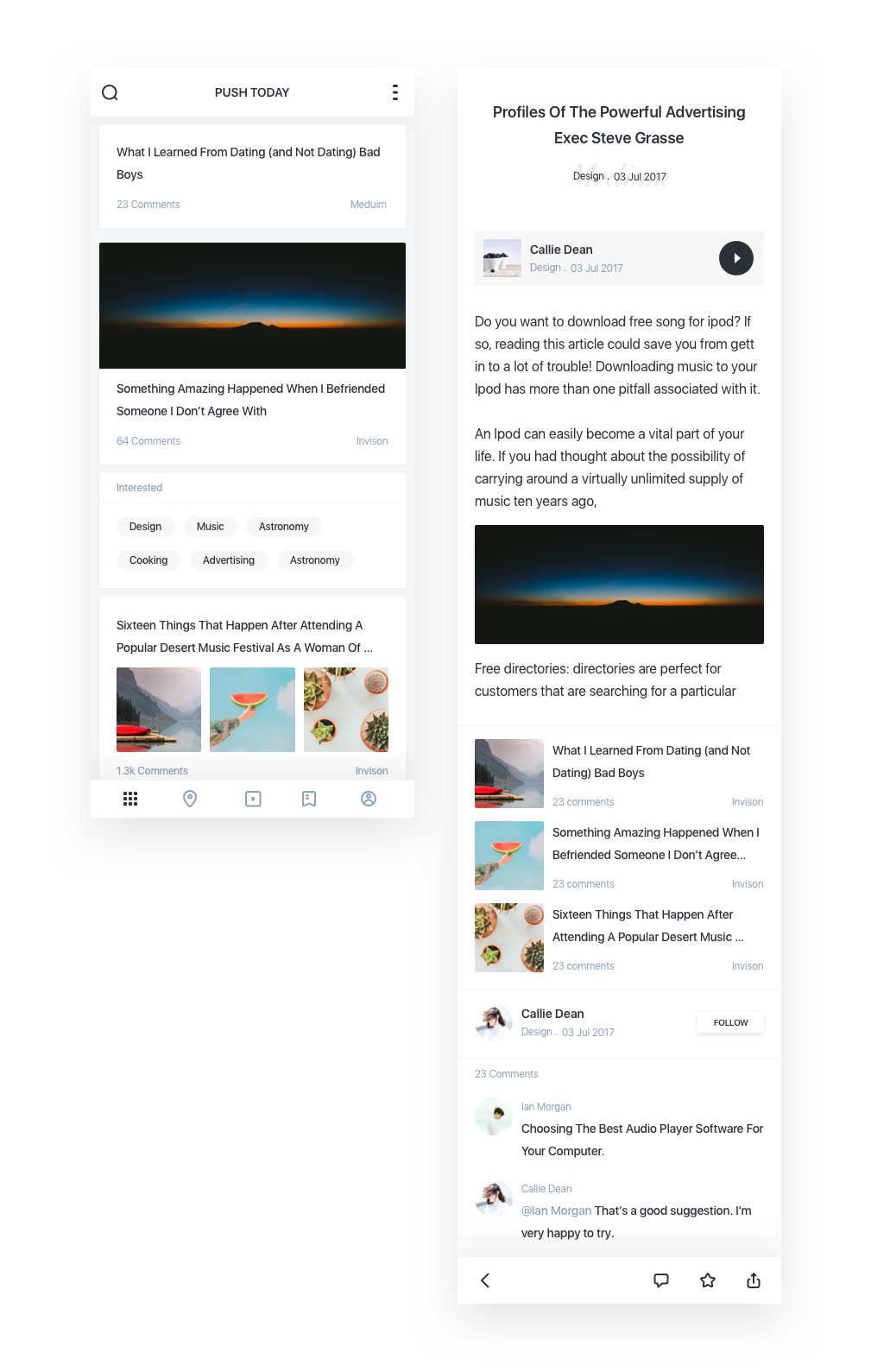The image consists of two side-by-side photographs, with the left photo being smaller. In the top left corner, there's a white box containing the text "Push Today". Adjacent to this, on the left, is a search icon, while on the right, there are three horizontal lines symbolizing a menu.

Immediately below this is a section displaying an article titled "What I Learned from Dating and Not Dating Bad Boys," enclosed in a box, with an interaction count showing 21 comments. Beneath this, another article titled "Something Amazing Happened When I Befriended Someone I Don't Agree With" is also situated in a noticeable box, showing it has 64 comments and is labeled as "Trending".

Further down, there is a partially legible title of another article, referencing "things that happened" followed by "blah," with accompanying images.

On the right-hand side, a more extensive white box presents an article titled "Profiles of the Powerful: Advertising Exec Steve Grassi". Below this, a gray box features what appears to be a music player with the prompt "Do you want to download a free song for iPod?". This section includes a photo similar to the sunrise or sunset image present on the left and features a different article title.